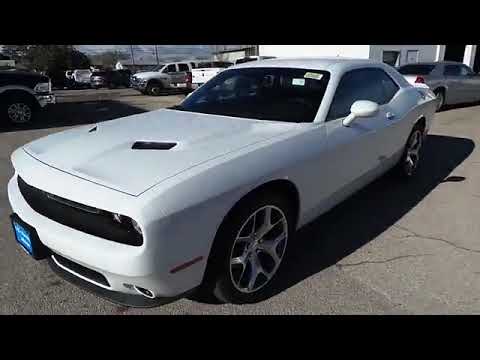The image depicts a modern white sports car with sleek, high-performance features, prominently positioned in a cracked gray cement parking lot. The car closely resembles a Mustang or possibly a Dodge Challenger from around 2008, identifiable by its iconic hood shape and dual-door design. The vehicle boasts an aerodynamic spoiler, fancy silver-patterned wheels, and distinctive root scoops. This car is likely a dealer vehicle, given the dealer plates, windshield stickers, and blue license plate background indicating it might be new. 

In the background, a few other vehicles, including trucks and a silver sedan, are noticeably parked near a white rectangular structure, suggesting a typical car lot setting. The photograph was taken during the day, evidenced by the car’s short shadow, implying a midday time frame. The image captures the sports car at an angle that emphasizes its dynamic design and polished exterior, against the more utilitarian setting of the surrounding parking lot.